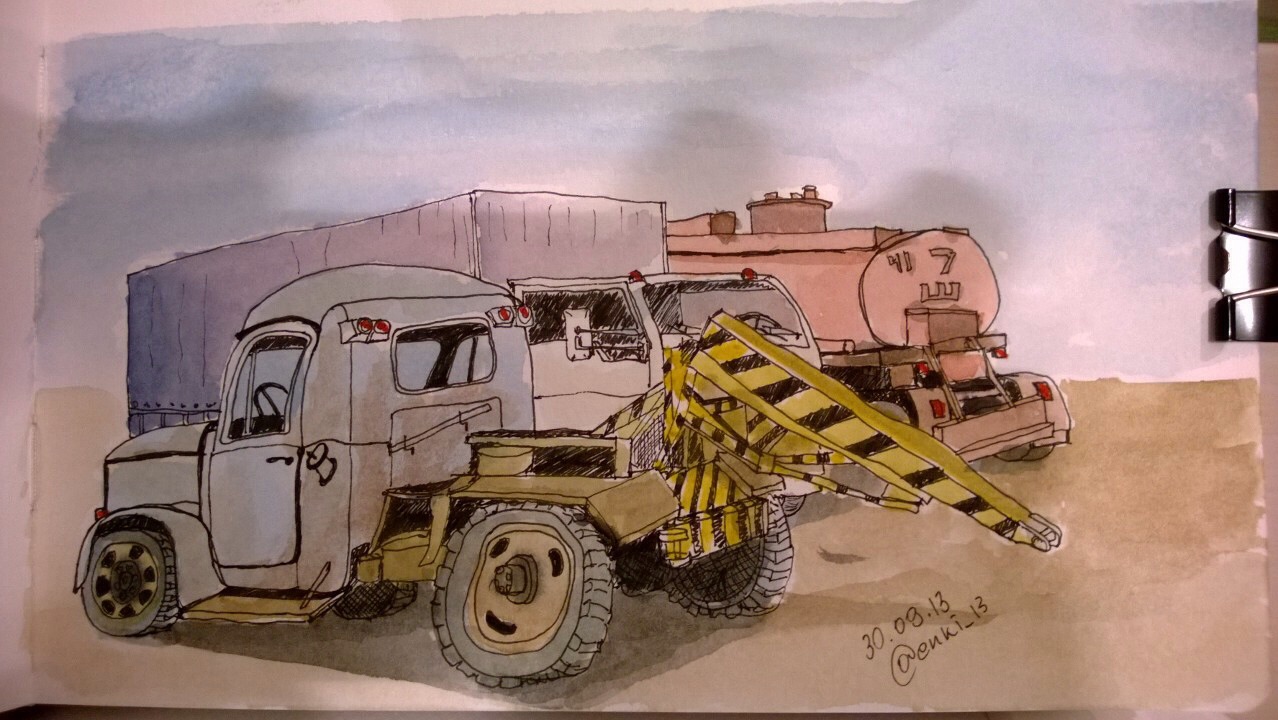This detailed watercolor drawing, secured by a black plastic and metal clip on the upper right, is presented on a paper with a subtle pink tint. The landscape features a clear blue sky above a light brown, sandy terrain. Prominently, an old-fashioned tow truck from the 1940s or 50s takes the foreground with its blue cab, massive black wheels, and a yellow and black striped lift on the back. Adjacent to this tow truck is a gray moving truck with a blue rear and white front. Further back, a tan tanker truck, possibly for gasoline, is visible with its cylindrical shape. The artwork is signed at the bottom right corner with an illegible signature and the date "30.08.13," accompanied by the text "Add" and the obscure markings "41.7" and "an upside-down E."